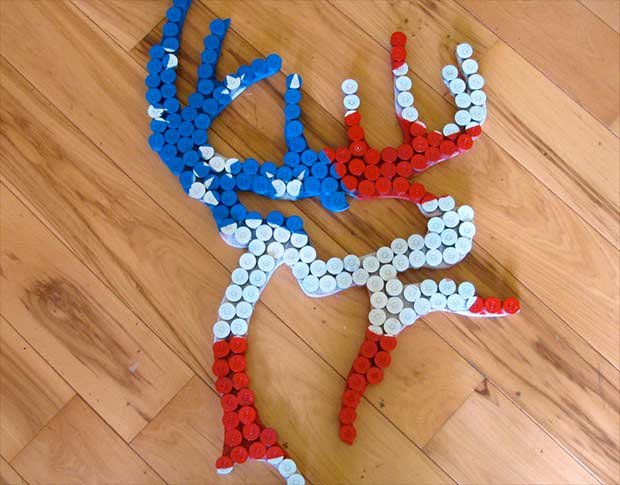On a light-colored wooden floor, there lies an abstract decorative piece composed of small, circular, plastic objects in red, white, and blue colors, reminiscent of the American flag. The upper left section features a cluster of blue circles with scattered white star-like patterns, while the rest of the piece includes irregular interpretations of red and white stripes. The formation, resembling a stag with prominent antlers, branches into six or seven paths on top and four on the bottom, creating a visually complex, almost vein-like design. The arrangement conveys an intricate and interpretive fusion of patriotic elements within an abstract, antlered animal figure, possibly a deer, crafted from these small, round components.